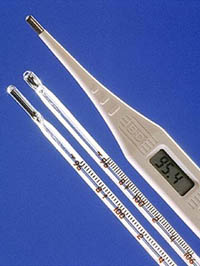A small, upright rectangular image features a deep blue background reminiscent of a clear, cloudless sky. Centered within the image are three different types of thermometers. The first is a modern white digital thermometer with a silver tip and a small window displaying the number "95.4," indicating a body temperature reading. Accompanying it are two classic glass thermometers filled with mercury. Each has a distinct design: one with a small bulb tip and the other with a slightly elongated cylindrical tip. These traditional thermometers display temperature readings on their sides, marked with lines and numbers starting from 96°F and extending up to 106°F, resembling precise measuring sticks made of glass.